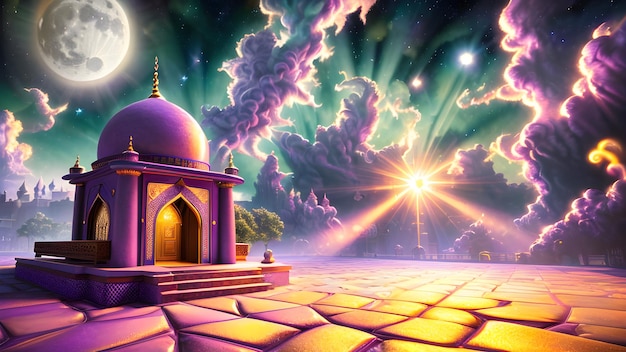This image appears to be a computer-generated print or oil painting depicting a fantasy world with an architectural structure reminiscent of a small temple or mosque, characterized by its minareted domed top and square bottom. The structure, located on the left side of the image, predominantly features purple hues with hints of gold and brown, including an orange door likely highlighted by reflections from the golden sun. 

A walkway made of reddish rose and gold-colored stones lies in the foreground. The sky, stretching across the background, is a kaleidoscope of purple and green with swirling clouds. A full moon occupies the upper left portion of the image, while a radiant sun illuminates the right side, contributing to the surreal and otherworldly ambiance. This detailed and vibrant scene evokes a sense of an animated video game environment or a fantastical dreamscape.